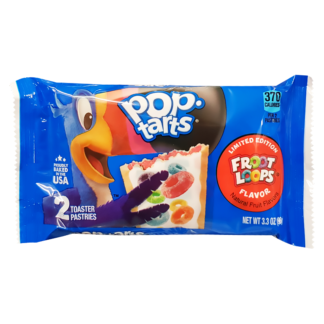The image depicts a centrally positioned package of Limited Edition Froot Loops Pop-Tarts, set against a stark white background. The wide, rectangular packaging is made of bright blue plastic and features white spikes on its edges. Prominently displayed on the left side is a vivid cartoon of Toucan Sam, characterized by a large beak colored in yellow, red, pink, and black, with the toucan itself adorned in bright blue and purple hues. Over Toucan Sam's beak, the words "Pop-Tarts" are written in white font, surrounded by a blue background. Additionally, Toucan Sam's arm holds a partially eaten Pop-Tart with white icing and multicolored Froot Loops—red, green, yellow, and blue—embedded in it. An orange circle on the right side of the package announces the "Limited Edition Froot Loops Flavor." The top right corner indicates the caloric content as 370 calories, and the bottom right corner notes the net weight of 3.3 ounces. The design, colors, and positioning suggest this could be a stock image typically seen on a supermarket website.